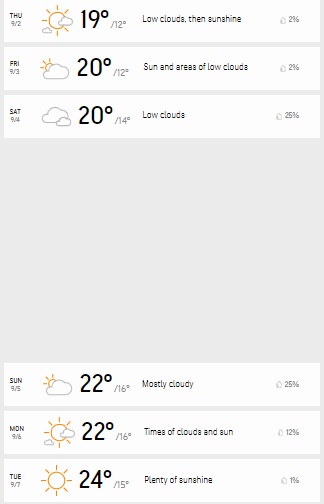**Detailed Weather Forecast**

**Thursday, 9/2:**
- **Weather Summary:** Low clouds transitioning to sunshine.
- **Temperature:** High of 19°C, low of 12°C.
- **Additional Details:** Partly cloudy with a 25% chance of either light rain or a gust of wind.

**Friday, 9/3:**
- **Weather Summary:** Sun with areas of low clouds.
- **Temperature:** High of 20°C, low of 12°C.
- **Illustration:** Larger cloud with the sun behind it.

**Saturday, 9/4:**
- **Weather Summary:** Predominantly low clouds.
- **Temperature:** High of 20°C.
- **Illustration:** Two clouds.

**Sunday, 9/5:**
- **Weather Summary:** Mostly cloudy with some sun peeking through.
- **Temperature:** High of 22°C.
- **Illustration:** Cloud with the sun partially visible.

**Monday, 9/6:**
- **Weather Summary:** Times of clouds and sun.
- **Temperature:** High of 22°C.
- **Illustration:** Mainly sunny with two tiny clouds.

**Tuesday, 9/7:**
- **Weather Summary:** Plenty of sunshine.
- **Temperature:** High of 24°C.
- **Illustration:** Full sun.